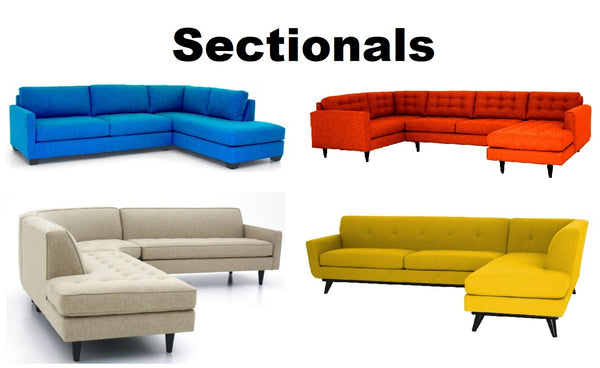This photograph showcases an arrangement of four distinctive sectional sofas, each in a different color and style, under the bold black title 'Sectionals' centered at the top of the image against a white background. 

In the top left corner, there is a royal blue L-shaped sectional sofa without visible legs, featuring back cushions and an armrest on the left-hand side. Directly to the right, the top right section houses a retro-inspired U-shaped sectional in a vibrant rust or orange color, characterized by tufted back pillows, high backs, and armrests flanking both sides, with a protruding section without an armrest. 

The bottom left corner displays a beige or tan L-shaped sectional with visible legs, a tufted cushion seat, a plain back, and an armrest on the right-hand side. Lastly, the bottom right showcases a retro yellow-gold L-shaped sectional, reminiscent of 60s or 70s appliances, featuring a high tufted back, plain cushions without tufting, visible legs, and an armrest on the left side.